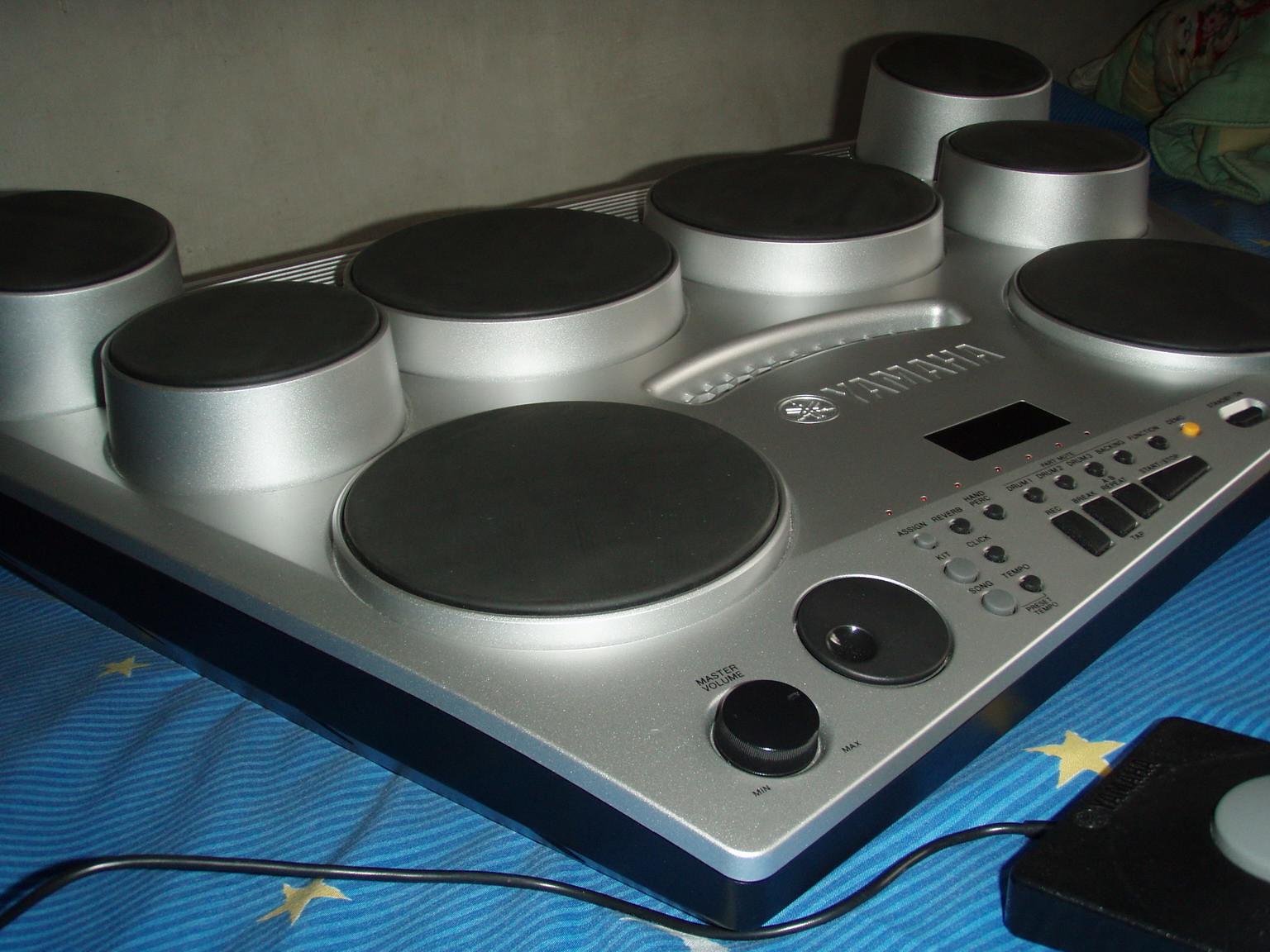This photograph showcases a Yamaha electronic drum set prominently placed against a white wall, which appears slightly dirty or beige. The drum set is primarily silver, featuring a black base with black drum heads, buttons, and knobs. The central panel of the drum set displays the Yamaha logo, with various buttons labeled "assign," "revert," "kit," "clip," "song," "tempo," and "rec," along with a knob marked "master volume" indicating max and min levels. Towards the bottom right, a black cord connects to a small black box with a gray button on top, hinting at additional control functions. The entire setup rests on a blue fabric adorned with thin, darker blue stripes and gold stars outlined in white. In the upper right corner, there is a green fabric featuring an animal face, adding a whimsical touch to the scene.